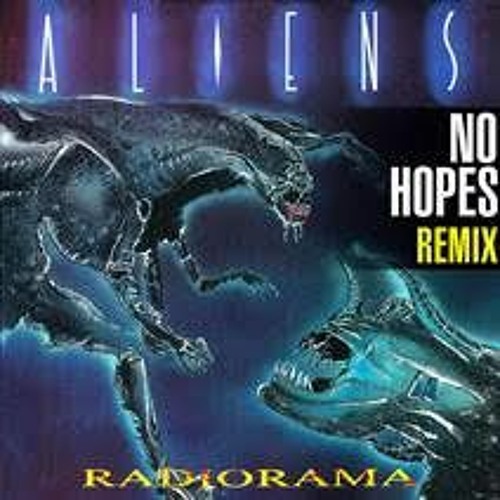The image appears to be a blurry, pixelated album cover or graphic inspired by the movie "Aliens." Dominating the top of the image is the word "Aliens," written in the iconic movie font with a bluish glow surrounding each letter. Against a dark bluish-black backdrop, two aliens are depicted in combat—one can be seen in the left-hand corner while the other is in the bottom right-hand corner. These creatures are characterized by sharp teeth, a bluish-green color, small heads, and several arms, reminiscent of the terrifying monsters from the film. To the right side of the image, bold white text reads "No Hopes Remix," with the word "Remix" highlighted in yellow. At the bottom of the image, the text "Radiorama" appears in yellow, which could likely be the artist's name.